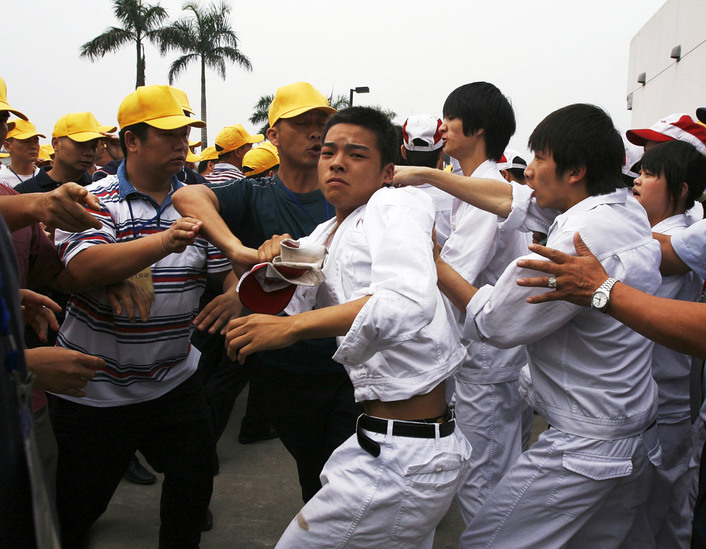The image captures a tense confrontation between two groups of men of Asian descent. On the right-hand side, a group of men all dressed uniformly in white pants and long-sleeve white jackets are being restrained as they clash with another group. The men on the left-hand side are characterized by their yellow baseball caps and diverse, colorful clothing, with some wearing white and red and blue striped shirts. A palpable sense of anger is evident on both sides as they yell and confront each other. One notable moment in the center of the group shows a man in a yellow hat pulling on the sleeve of a man in a white jacket. The backdrop features a white sky, several palm trees, and part of a white building on the right. The atmosphere is charged, with individuals pushing and shoving, indicating that a fight is erupting.